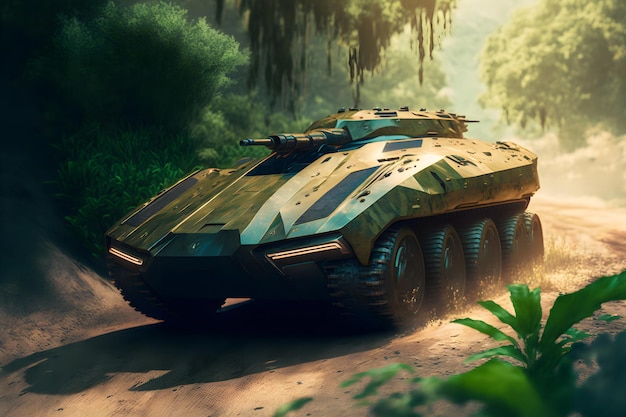This detailed digital rendering of a futuristic armored personnel carrier (APC) showcases it traveling along a curved, flat dirt road in a lush jungle setting. The APC, covered in a camouflage pattern of greens and lighter greens, features five thick black wheels on each side. Its body is accented with beige tones to signify depth and shadows. A small, black cylindrical turret protrudes from the top hatch. In front of the APC, a green plant is visible, adding to the dense vegetation which includes mossy substances hanging over the tank. A green cluster of leaves appears in the right corner, suggesting rich foliage characteristic of a rainforest. In the background, more green vegetation and rainforest-style trees frame the scene, with some branches overhanging the APC, resembling the drooping leaves of a weeping willow. As the APC moves, it's seen kicking up dirt behind it, with particles cascading along the road, emphasizing its motion. The entire setting suggests a daytime operation amidst the dense and vibrant flora of a jungle environment.